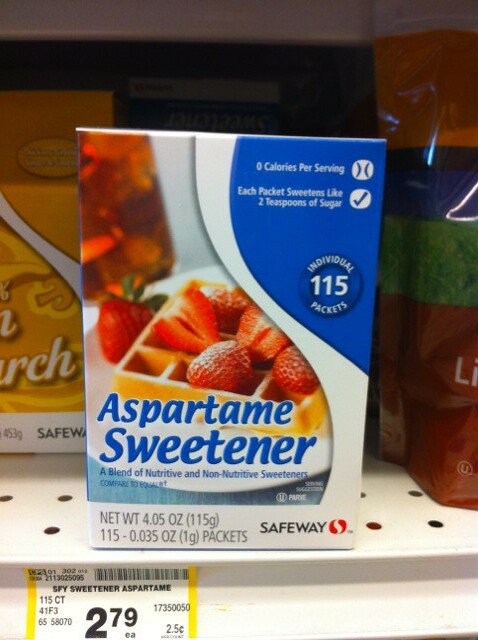This image captures a boxed product prominently displayed on a grocery store shelf. The box, featuring a color scheme of white, red, and blue with accents of black and white print, is labeled "Aspartame Sweetener" in bold blue letters. The top right corner of the box is marked with a blue area highlighting key product details in white print: "Zero Calories Per Serving" and "Each Packet Sweetens Like Two Teaspoons of Sugar." Beneath this, the text specifies the contents as "115 Individual Packets."

To the left side of the box, an appetizing image shows a beige waffle topped with fresh red strawberries placed on a clean white plate, set against a white background. The box is positioned on a typical grocery store shelf, characterized by its sturdy, heavy steel construction with punched holes and an off-white color. Below the box, there's a white shelf label bearing the price, $2.79, along with additional product information.